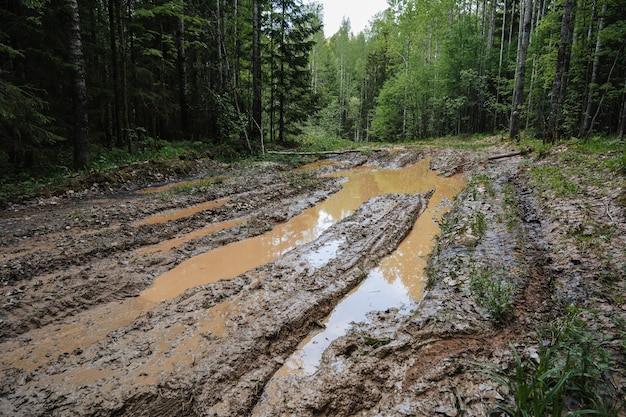Set amidst a dense, vibrant woodland, the image captures a rugged four-wheeling or logging trail dominated by a giant mud pit. The trail, lined by imposing trees with gray trunks and thick, green foliage, is muddied with dark brown, chocolate milk-colored water, creating deep ruts and tracks from passing vehicles. The mud hole appears extensively churned, with rows of tire marks forming across its length. Patches of grass sporadically sprout among the puddles and muddy paths. The entire scene is encased by lush greenery, with pine trees and green grass flanking the left side and a thick, dark forest background stretching throughout. The mud pit is most profound at its center, with visible muddy water marking the submerged tracks. The overall picture is a chaotic blend of mud, water, and foliage, highlighting the trail's harsh, untamed nature.